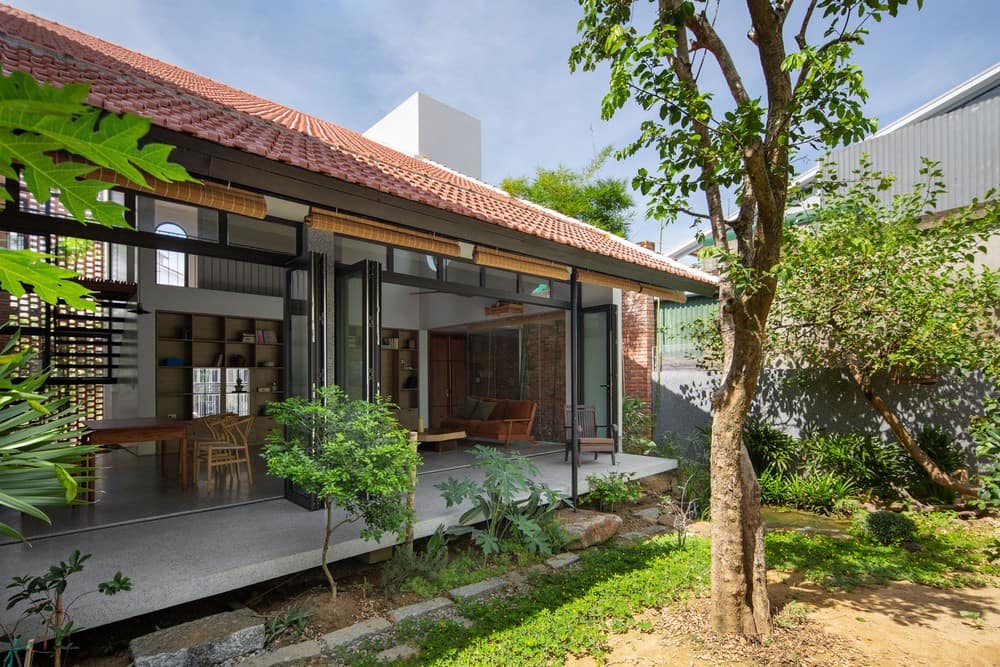The picture showcases the exterior of a beautiful, one-and-a-half-story tropical home. The vibrant blue sky and glimpses of white clouds serve as a picturesque backdrop. The house features a distinctive red ceramic tiled roof and large glass folding doors that open out into a lush courtyard. In the courtyard, patches of green grass and several small trees, including a split-leaf philodendron, create a serene natural atmosphere. To one side, there is an additional building, which might be part of the residence or a meeting place. The area is adorned with a little garden of thriving green plants. The home’s interior, visible through the expansive glass doors, includes a cozy living room with a brown table, light brown chairs, a dark orange sofa, a coffee table, and numerous bookshelves. Inside, a set of stairs lead to the second floor, emphasizing the spacious and inviting layout of this tropical retreat. A covered porch, shaded by the extending roofline, and a white chimney add to the architectural charm of this idyllic getaway.